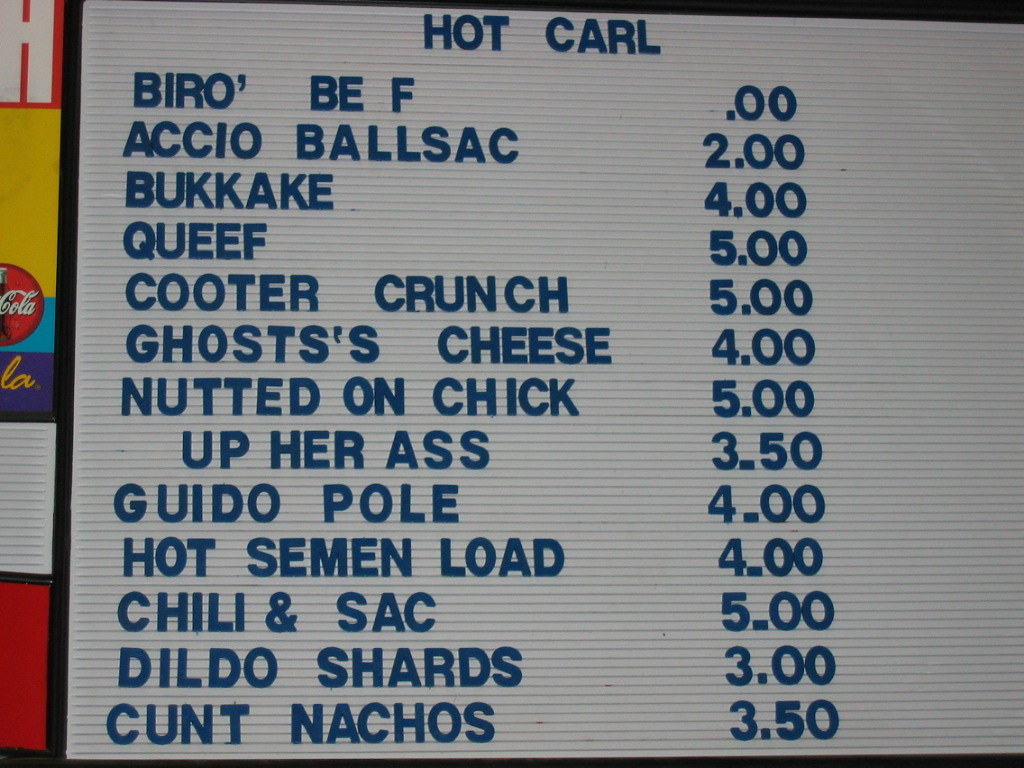The image features a white board prominently displaying a menu for a restaurant named "Hot Carl." The letters and numbers on the board are in blue against the white background, making them stand out clearly. The menu includes a variety of intriguingly named items, each with its corresponding price. The list begins with "Burro Beef," indicating the type of beef used. Following this are:

- "Accio Balsak" priced at $2
- "Bouquet" priced at $4
- "Cueef" priced at $5
- "Cooter Crunch" priced at $5
- "Ghost Cheese" priced at $4
- "Nutted on Chick" priced at $5
- "Upper Ass" priced at $3.50
- "Guido Pole" priced at $4
- "Hot Semen Load" priced at $4
- "Chili and Sack" priced at $5
- "Dildo Schnards" priced at $3
- "Conked Nachos" priced at $3.50

The names of the food items are quite unusual and provocative, leaving one to wonder about the nature and flavors of these offerings.